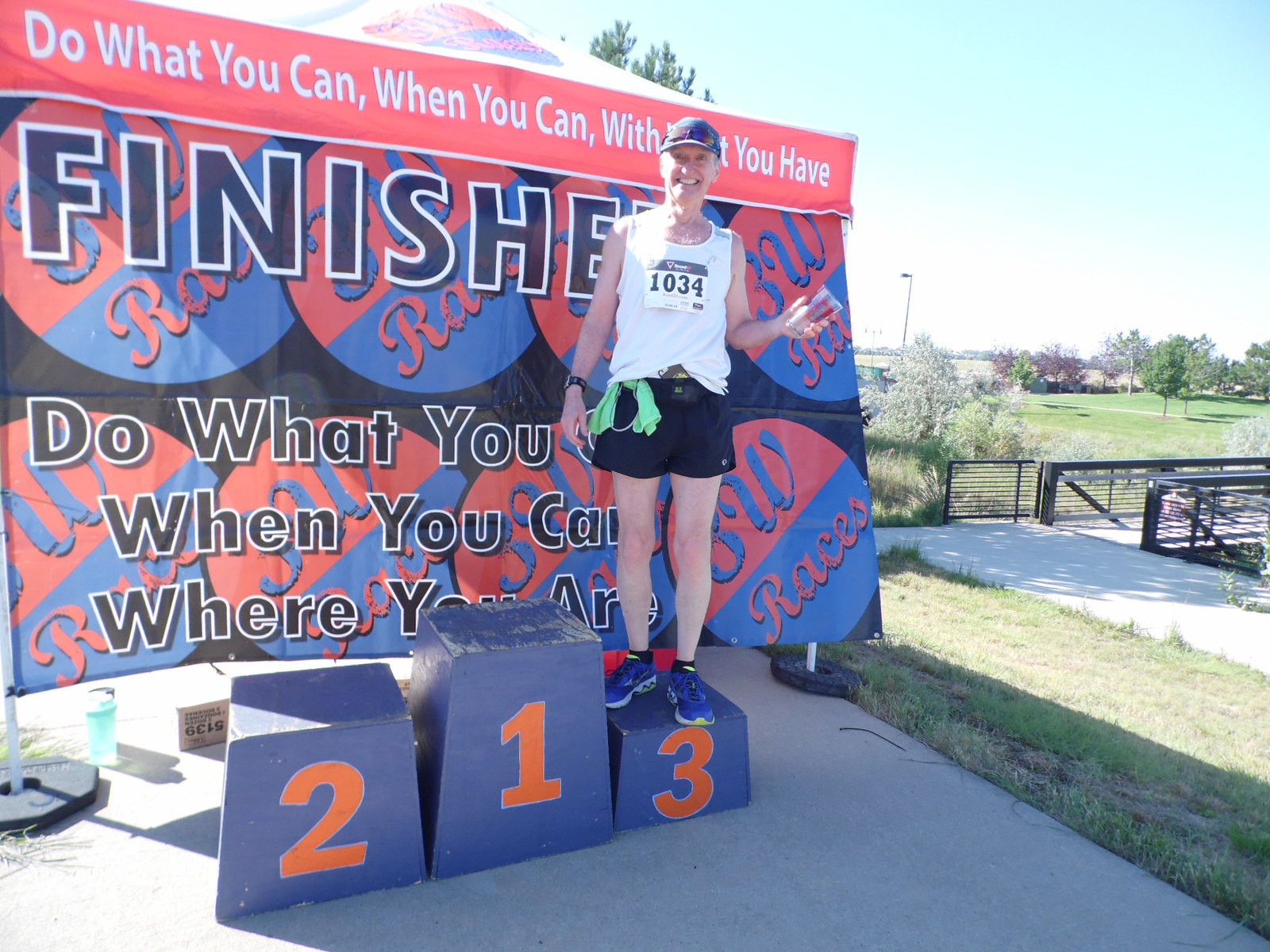In this outdoor photograph, a man who appears to have just finished a race is standing proudly on a set of three blue podiums marked with the numbers 1, 2, and 3 in orange. He occupies the podium marked with the number 3. The man is dressed in a white tank top with the race number 1034, black shorts, blue running shoes, and a blue baseball cap with sunglasses resting on top. He is smiling and holding a glass in his left hand. Sunlight softly illuminates his face, while the rest of his body remains in the shade. Behind him, a large banner displays the motivational phrases: "Do what you can, when you can, with what you have." and "Do what you can, when you can, where you are," along with the word "finished" and some circular logos that likely read "SW Races." The background features a clear, light blue sky, a pathway with a metallic bridge, and a lush green landscape of grass, trees, and lampposts. There are no other people visible in the scene.